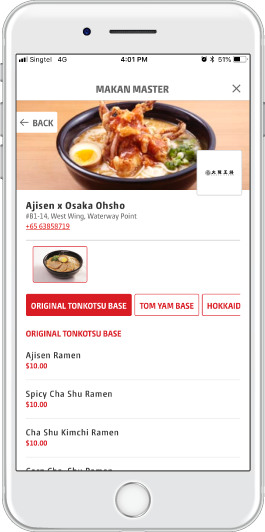The image shows a silver or white iPhone, identifiable by three buttons on the left side, one button on the right side, and a circular home button at the bottom. At the top of the screen, the display reads "SyncTel 4G" in black text on a white background, with the time showing 4:01 p.m. An alarm clock icon is present but appears blurry. Next to it, the battery percentage reads either 51% or 61%, followed by a battery icon in black.

Below this status bar, there is a section labeled "MAKAN Master" with a gray 'X' next to it. The primary image underneath depicts a black bowl containing what seems to be a halved boiled egg, green scallions, and possibly bacon. The description is somewhat unclear, particularly about the topping near the top section of the bowl. 

Adjacent to this image, there's a gray rectangle and directional text, with a black arrow pointing right, followed by the word "back." Directly below, the text "Agilson" is displayed, indicating an "ex-Osaka HOSHO," located at "B1-14 West Wing Waterway Point." The phone number "6563 858 719" is highlighted in red. The menu details various options: "Original Tonkotsu Base" and "Tom Yum Base." It lists different ramen varieties such as "Agilson Ramen" in black text and "Spicy Char Siu Ramen" and "Char Siu Kimchi Ramen," both priced at $10 and highlighted in red.